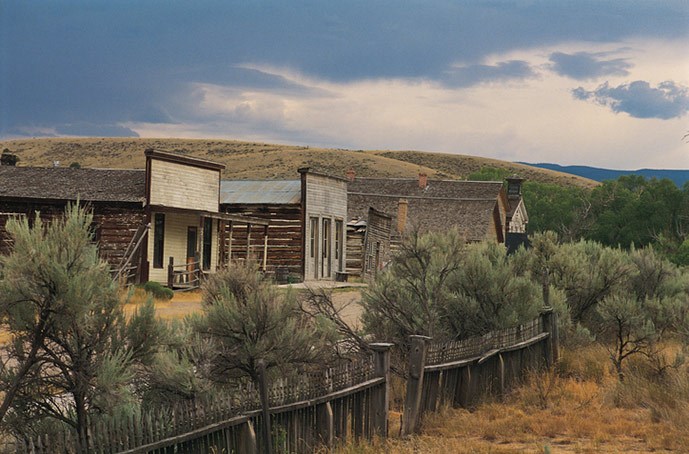This evocative photograph captures the ambiance of an Old West town, reminiscent of a ghostly movie set. A dusty dirt street, lined with approximately four to five wooden structures, stretches from the center left edge to the center and slightly right, forming a diagonal line. These weathered buildings, possibly erstwhile general stores or lodgings, bear no signage aside from rectangular spaces hinting at bygone displays. The scene is arid yet punctuated with patches of green shrubbery and mesquite bushes. In the foreground lies an old wooden fence with barbs, interrupted by a gap and tapering off into thick green underbrush. Towards the bottom right corner, the ground is a mix of orange-hued grass and soil. Behind the town, rolling green hills rise toward a cloudy, overcast sky, embedding this seemingly abandoned Western settlement in a timeless, picturesque landscape.